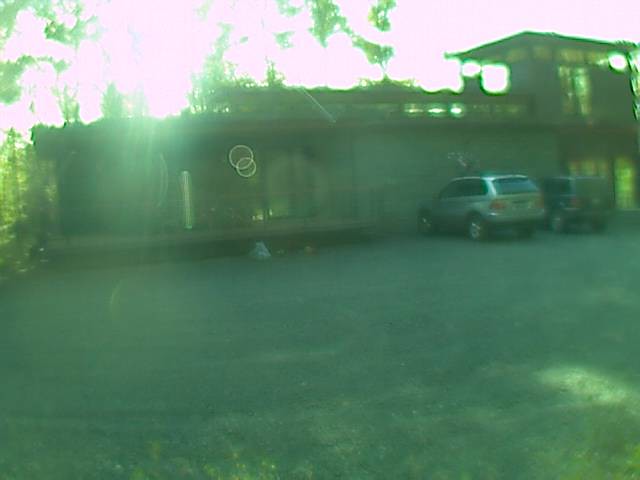In this bright image, the sky occupies a significant portion, with a noticeable glare in the top left corner, casting multiple lens flare circles toward the center. Dominating the middle section is a long building, slightly elevated from the ground, with a garage or entryway prominently featured. The top right of the building reveals a larger structure, likely made of glass. To the right, two cars are parked: a silver car closest to the building and a black car beside it. The foreground consists of a dirt road with dappled sunlight in the bottom right. On the far left, a few trees can be seen, adding a touch of greenery to the scene.